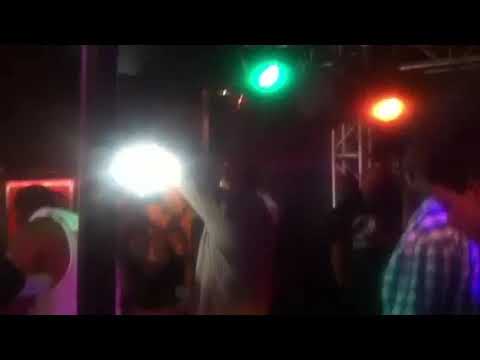In this dark, nighttime concert photo, the stage is illuminated by three prominent spotlights that stand out against the obscured background. A white light on the left, a higher green light in the middle, and a red light on the right cast an ethereal glow over the scene. The image reveals faint figures of about four to five people mulling around, though their details are indistinct due to the dim lighting and light-induced fuzziness. On the lower right corner, there is a partially visible profile of a person in a plaid shirt, suggesting it's a side view of a man. Behind the figures, some metallic scaffolding hints at the stage setup. Despite the photo's darkness and the difficulty in discerning finer details, the spotlights and the scattered individuals evoke a lively, albeit shadowy, concert atmosphere.